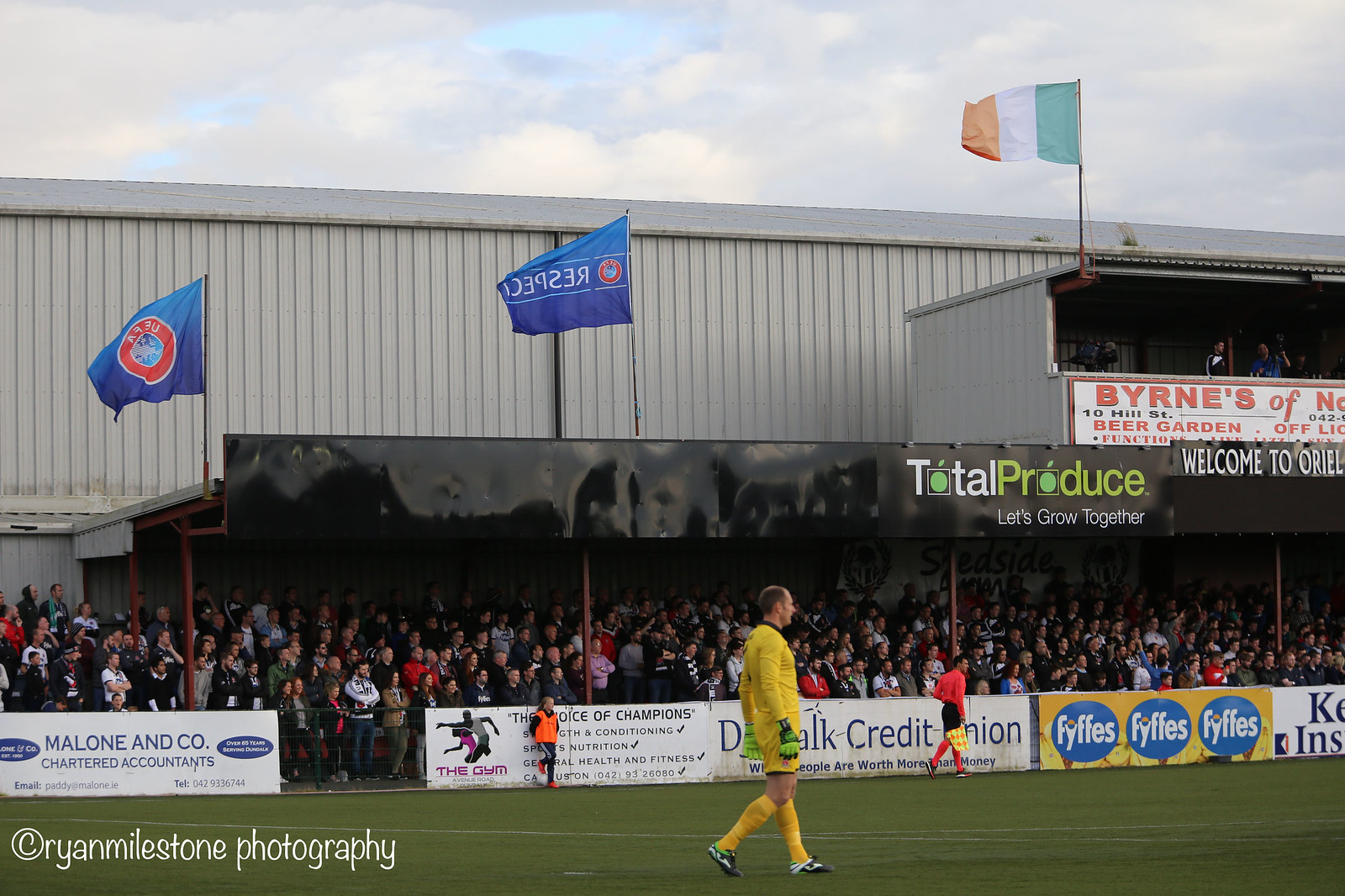This detailed photograph captures a soccer match in progress under a cloudy sky at a large, fully packed stadium. The scene is bustling with spectators, all of whom are intently focused on something off to the right side of the image. The audience, seated under a covered grandstand, stands behind a fence adorned with various advertisements, including those for Total Produce with the slogan "Let's Grow Together," Credit Union, Malone and Company Chartered Accountants, and FYFFES. 

The perspective of the photo is at eye level, likely taken from the sidelines near the stands. In the foreground, a player in a bright yellow uniform, complete with long sleeves, shorts, and socks, is walking while looking towards the right side of the field. To his side, another player in an orange long-sleeved jersey, black shorts, and orange socks exhibits a similar posture. Both players are captured in profile, not running but walking towards one end of the field. 

In the background, an official or referee can be seen also looking rightward. The stadium’s infrastructure includes a grey, metallic building wall and an elevated, enclosed section that seems to cater to VIPs or press members. An Irish flag prominently flies at the center of the image, adding a touch of national pride to the scene. The bottom left corner of the photograph credits "Kryan Milestone Photography, C-R-Y-A-N Milestone Photography."